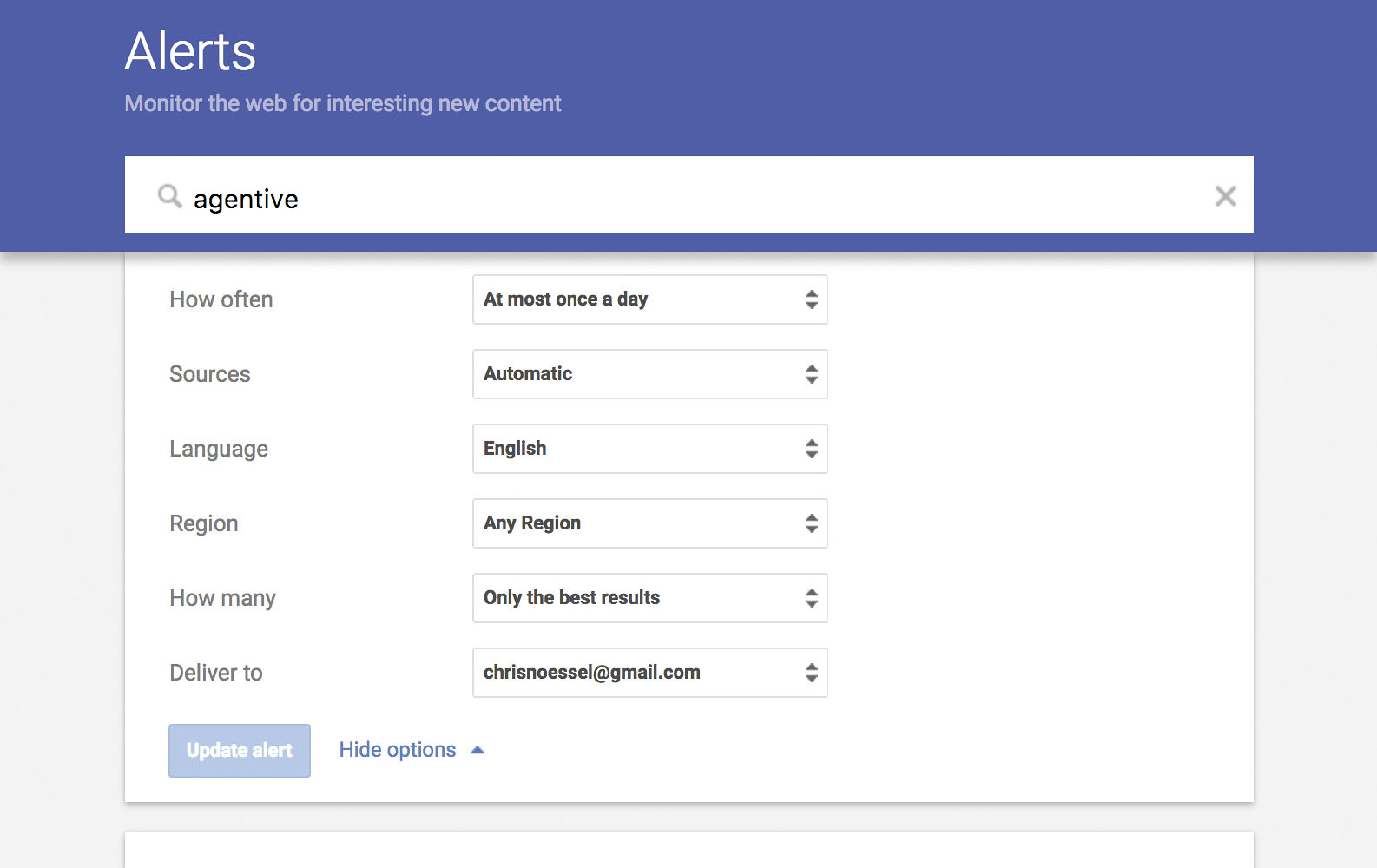The image displays a computer screen with alert settings. At the top of the screen, a long, lighter blue rectangle spans across with white text. On the left side, in bold, it reads "Alerts". On the upper right corner, in smaller white text, it says "Monitor the web for interesting new content." 

Beneath the blue rectangle lies a long, white search bar. On the left side of the search bar, there's a gray magnifying glass icon, followed by the black text "agentive." On the far right of the search bar is a small gray "X."

Below this, the background shifts to an off-white color containing a white drop-down menu. The first line of the menu reads "How often" on the left, with "At most once a day" on the right. Following this, the next line says "Sources" with "Automatic" on the right. Continuing, it lists "Language" followed by "English," then "Region" paired with "Any region," and "How many" with "Only the best results."

At the bottom of this section, it shows "Deliver to" followed by the email address "Chris Onessi at gmail.com." Finally, beneath all the other settings, there are two options: "Update alert" and "Hide options."